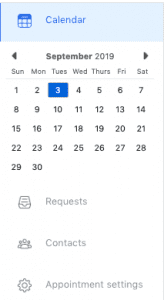The image depicts a blurry and low-quality photo of a digital calendar interface. At the top, there is a small blue calendar icon, followed by the word "Calendar" on a light blue banner. Below this, centered in black text, is "September 2019," flanked by left and right navigation arrows. The calendar grid displays all the dates of the month, with Tuesday, September 3rd highlighted in a blue box. Underneath the calendar, there are section headings in a very light gray font, labeled "Requests," "Contacts," and "Appointment Settings."